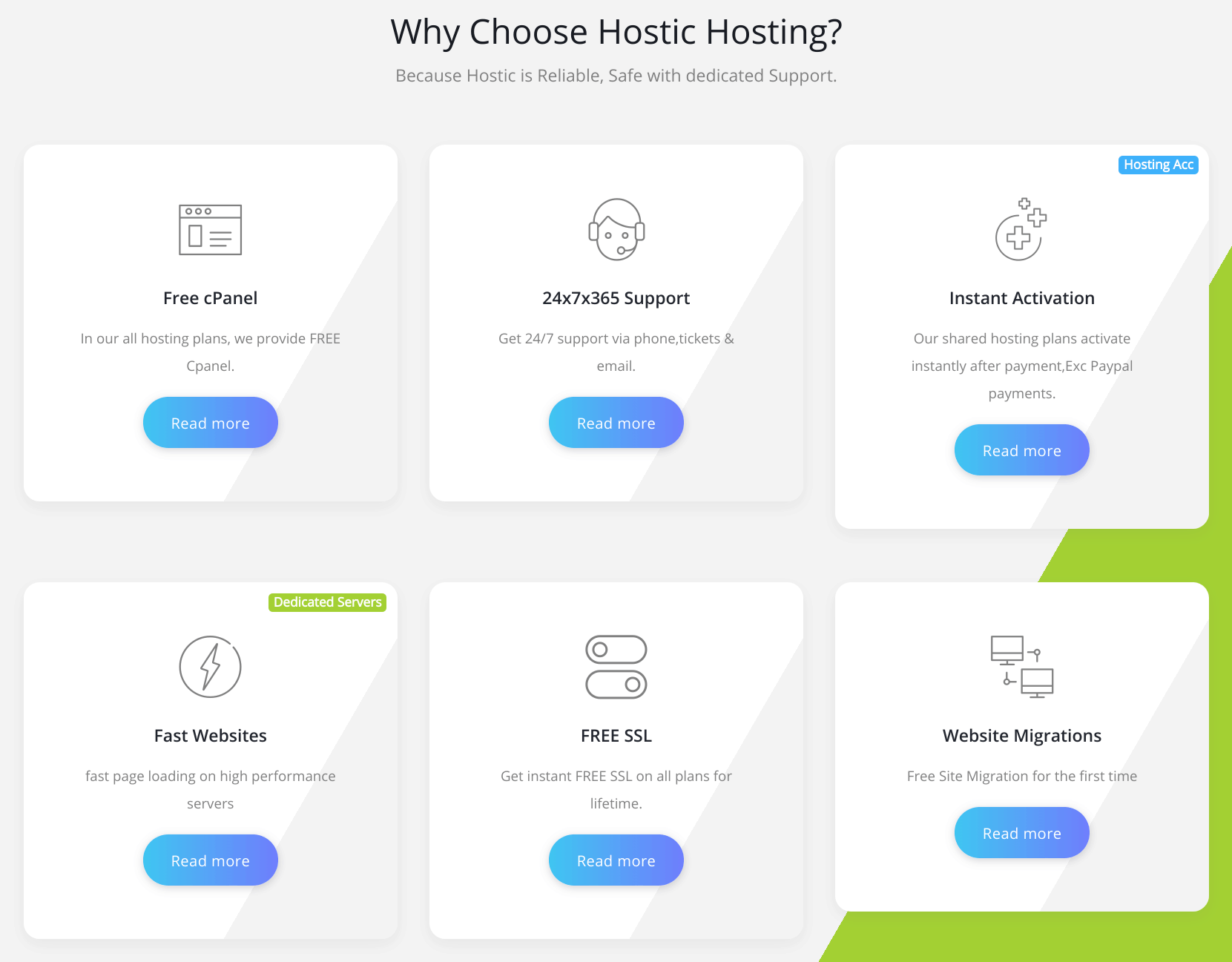The image features a promotional graphic by Holstic Hosting set against a light gray background. In the center, black text reads, "Why choose Holstic Hosting?" Below this heading, additional text states, "Because Holstic is reliable, safe, with dedicated support."

The image contains six outlined white boxes, each with a gray slanted section on the right side. At the bottom center of the image, a blue semicircle button with white text states, "Read More."

1. **Box 1:** 
   - **Top:** An icon featuring three dots, a square, and three lines.
   - **Title:** "Free cPanel"
   - **Description:** "In all our hosting plans, we provide free cPanel."
   - **Button:** Blue "Read More" button.

2. **Box 2:** 
   - **Top:** Icon of a person's head wearing headphones with a microphone.
   - **Title:** "24 x 7 x 365 Support"
   - **Description:** "Get 24/7 support via phone, tickets, and email."
   - **Button:** Blue "Read More" button.

3. **Box 3:** 
   - **Top:** Light blue box with "Hosting ACC" in white font, featuring three plus symbols with the largest in the center, encircled by a half-circle.
   - **Title:** "Instant Activation"
   - **Description:** "Our shared hosting plans activate instantly after payment, including PayPal payments."
   - **Button:** Blue "Read More" button.

4. **Box 4:** 
   - **Top:** Light green box with white text, "Dedicated Servers," and an icon of a circle with a lightning bolt.
   - **Title:** "Fast Page Loading"
   - **Description:** "Free websites, fast page loading on high-performance servers."
   - **Button:** Blue "Read More" button.

5. **Box 5:** 
   - **Top:** Digital on/off buttons.
   - **Title:** "Free SSL"
   - **Description:** "Get instant free SSL on all plans for a lifetime."
   - **Button:** Blue "Read More" button.

6. **Box 6:** 
   - **Top:** Icon of two monitors, one pointing at the other.
   - **Title:** "Website Migrations"
   - **Description:** "Free site migration for the first time."
   - **Button:** Blue "Read More" button.

The graphic also includes a small lime green triangle partially covering the bottom right corner of the final box.